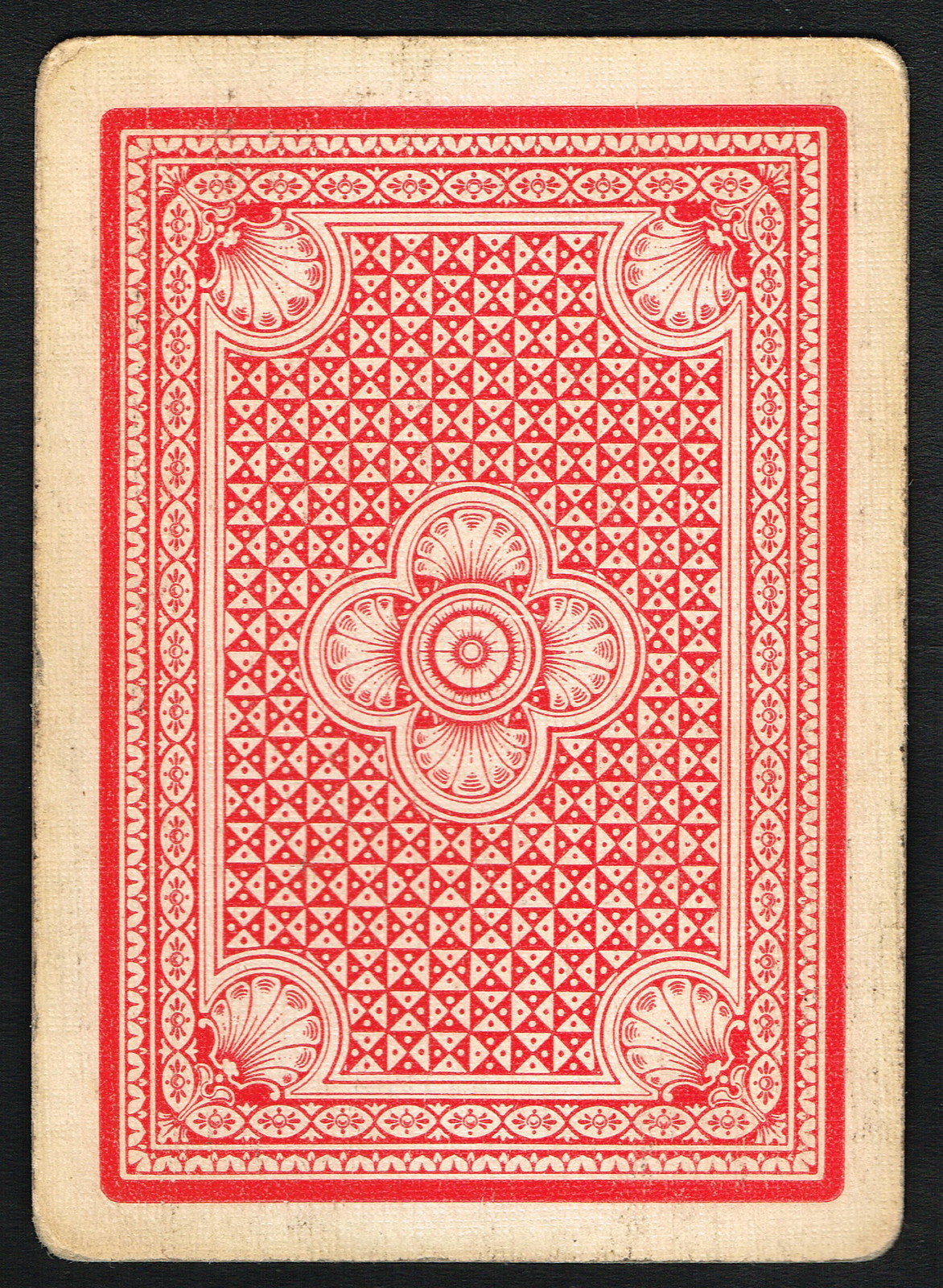This image showcases the back of a well-used playing card, likely from a casino set. The card's once-white surface has succumbed to the passage of time, now exhibiting significant grime and discoloration, especially around the corners and edges, giving it a distinct yellowish hue. The card appears to feature a crosshatch or grain pattern characteristic of a vinyl material, indicating it's of higher quality than standard paper cards.

The design on the back is intricately detailed, starting with an outermost red border. Within this boundary lies another red border adorned with semi-circles, followed by a third border decorated with an eye-like pattern, also in red. As we move further inward, there is a layer featuring seashell motifs. Finally, at the center of the card is a striking alternating checkered pattern composed of red and uncolored triangles, adding a vibrant focal point to the design.